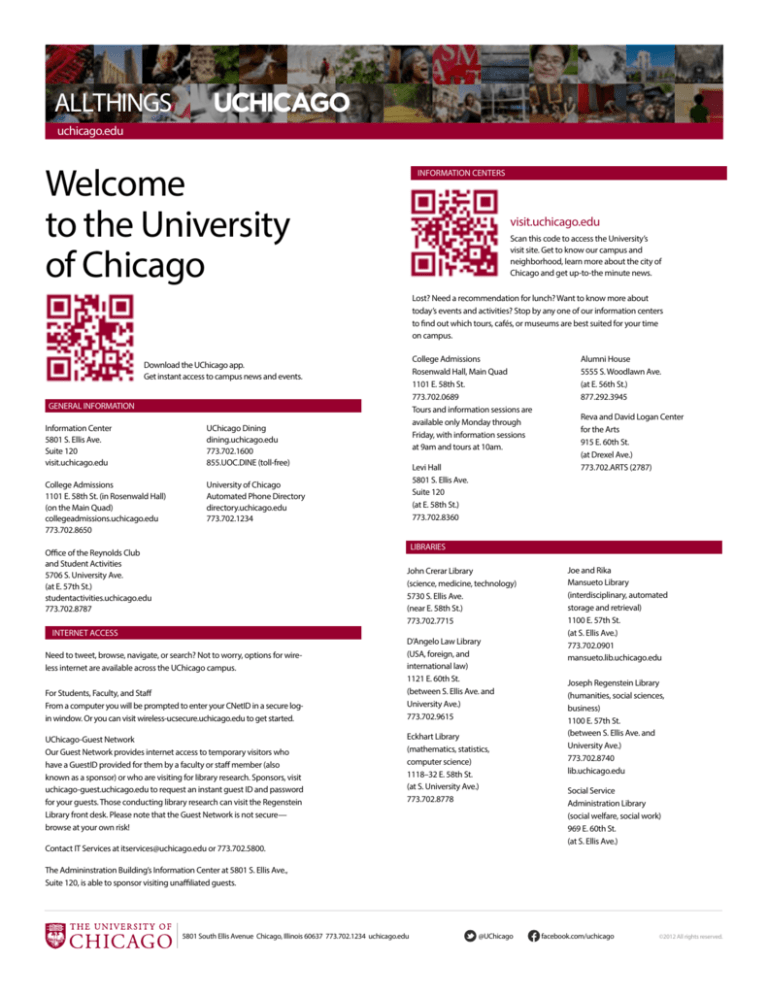This animation resembles a computer screenshot. At the very top, there's a header composed of numerous small square images, some showing people's faces while others appear to be random pictures. In the top left corner, there is text that reads "All Things UChicago." Below that, on the left side, there is a welcome message stating "Welcome to the University of Chicago," accompanied by a red QR code. 

Further down, a red heading is visible, including the word "General" with an adjacent word that is not legible. Below this heading are various informational options: Information Center, College Admissions, and Office of Reynolds Club. Another red heading appears, discussing topics related to internet access. Underneath it, there are several paragraphs containing detailed text information.

Returning to the top right, another red QR code can be seen, labeled "visituchicago.edu." Adjacent to this, a red heading lists the different libraries available on campus.